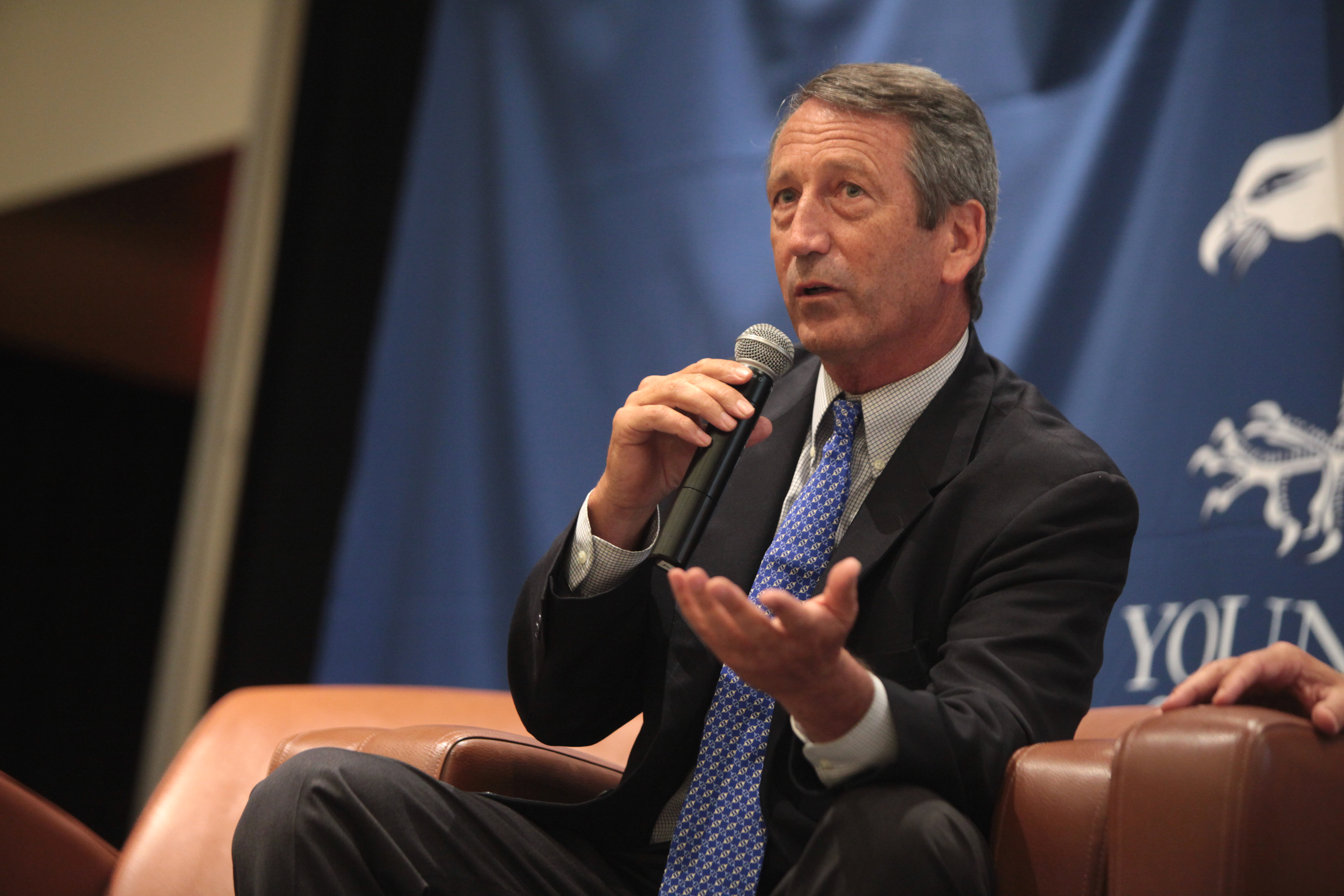This photographic indoor image captures a distinguished man in his 50s or 60s with short-cropped gray hair, seated in a brown upholstered leather chair. Dressed in a gray suit with a white or off-white shirt and a long blue tie adorned with white geometric designs, he holds a black microphone with a silver speaker close to his mouth. His right hand extends outward as if to emphasize his speech, and he looks slightly upward, engaging with his audience. Behind him, a blue banner featuring a partial graphic of a bird's head and claws, along with the partially visible letters "Y-o-u-n," forms the background. Additionally, a white person's hand rests on the side of the chair, adding a subtle detail to the scene.